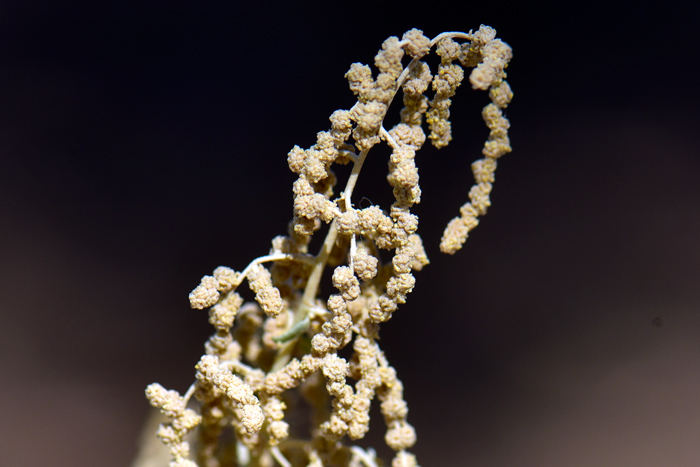This is a color photograph, presented in landscape orientation, that captures a detailed, dried ragweed-type plant. The plant curves elegantly from the bottom left of the image, leaning towards the upper right, and then bending back down with its top blossoms hanging. The plant’s central stem and multiple shorter branches are adorned with clusters of small, round flowers or seeds that resemble popcorn in shape, ranging from a light brown to a cream or beige color, with occasional faint green touches. The background of the image is predominantly black, creating a stark contrast that highlights the plant’s intricate details. The corners of the photograph, particularly the bottom ones, feature lighter gray areas that softly fade into the dark backdrop, adding depth to the composition. Overall, the photograph exhibits a photographic representational realism style, emphasizing the plant’s texture and form against the subtly varied background.